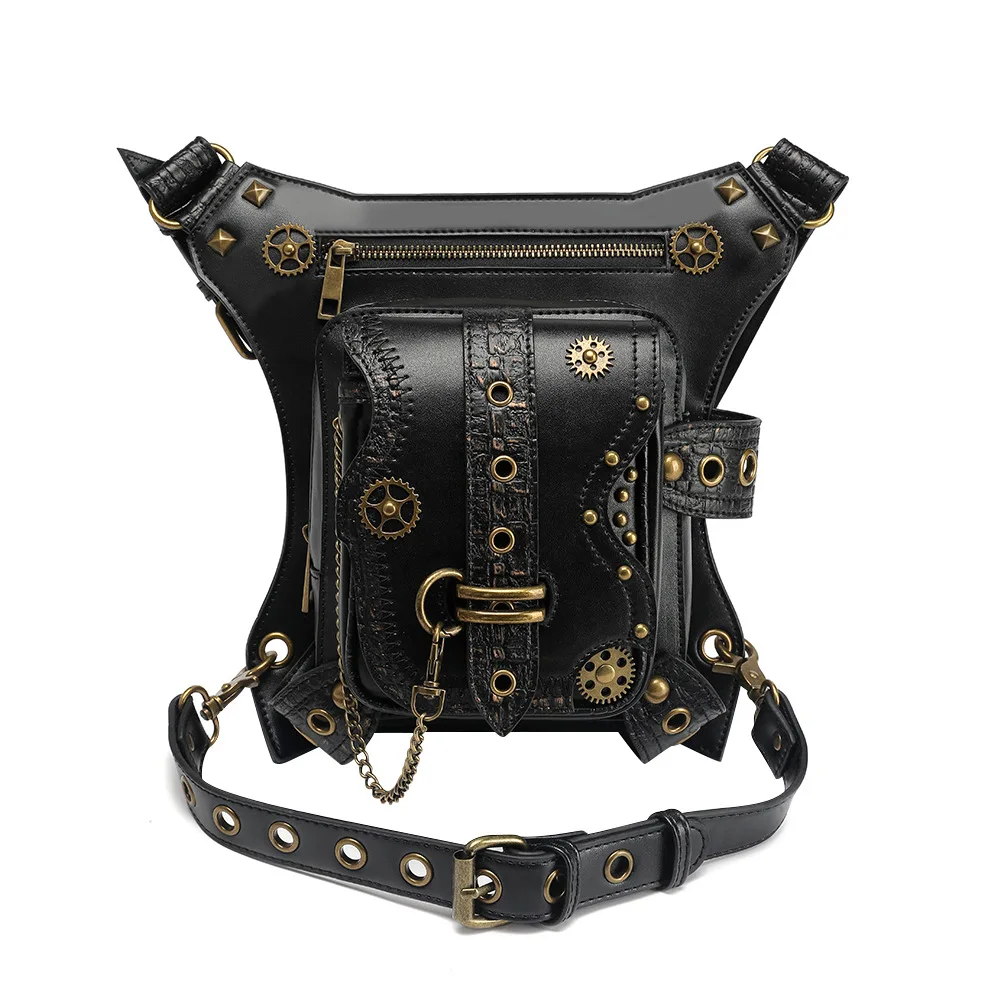This photograph displays a uniquely designed black leather bag, featuring a geometric and somewhat Y-shaped form at the top. Styled in steampunk fashion, it is adorned with brass-colored gears, chains, and other metal decorations. The bag includes multiple functional elements: at the top, there are two extended straps and a zippered pouch; farther down, the main body of the bag has a clasp running through its center, accompanied by extra clasps on the sides. At the bottom, an adjustable belt with several grommets and metal pieces completes the design, enhancing both its aesthetic and practical utility. The bag also features intricate black embroidery patterns sewn into the leather, adding to its distinctive appearance.